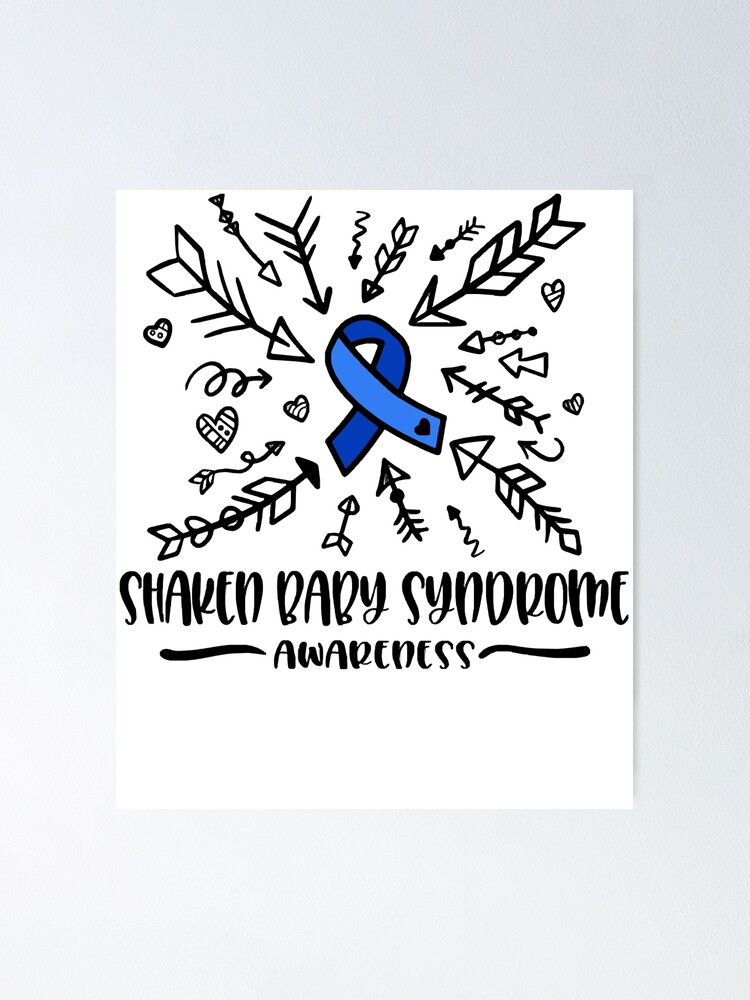The image is a color poster primarily in black and white, featuring a prominent blue ribbon with a darker blue heart on the lower right side, situated at the center of the composition. The background is predominantly white, with soft grey shading in the lower left and right corners. Surrounding the blue ribbon are various hand-drawn arrows in a mix of styles, including squiggly, curlicue, and straight arrows, all pointing toward the ribbon. Interspersed among the arrows are small hearts, some adorned with lines and dots. At the bottom of the poster, in bold black capital letters, it reads "Shaken Baby Syndrome Awareness," flanked on either side by thick, swirling lines. This intricate arrangement serves as a visual emblem to raise awareness about Shaken Baby Syndrome.